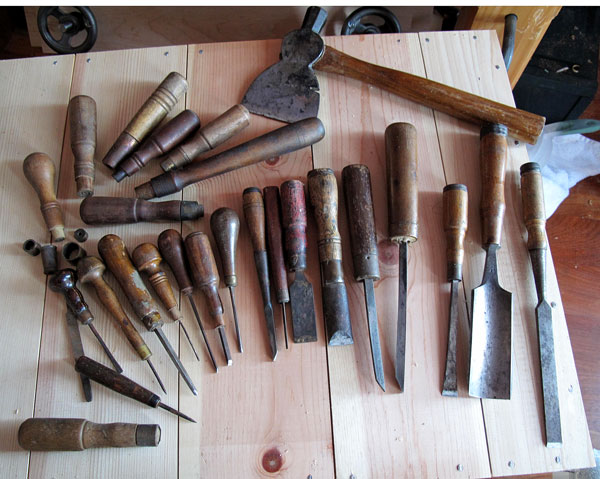The image captures a newly handcrafted wooden table made from unfinished planks, possibly pine, assembled with fresh nails giving it a sturdy appearance. On top of this table lies a diverse array of tools, neatly arranged in a workshop setting. Most tools, characterized by their wooden handles in various shades of brown and metal implements, are designed for different carpentry tasks such as cutting, chipping, and digging. Prominently, an axe is positioned in the upper right-hand corner of the table. Among the other tools are numerous awls and file-like implements, some orientated vertically, while others are placed diagonally, stretching from the upper left corner towards the center. The tools and handles vary in length and size, with some appearing to be either broken off or designed to be interchangeable. The table is set against a backdrop of partial images hinting at additional equipment, possibly indicating the ambiance of an active woodshop, bathed in natural daylight.